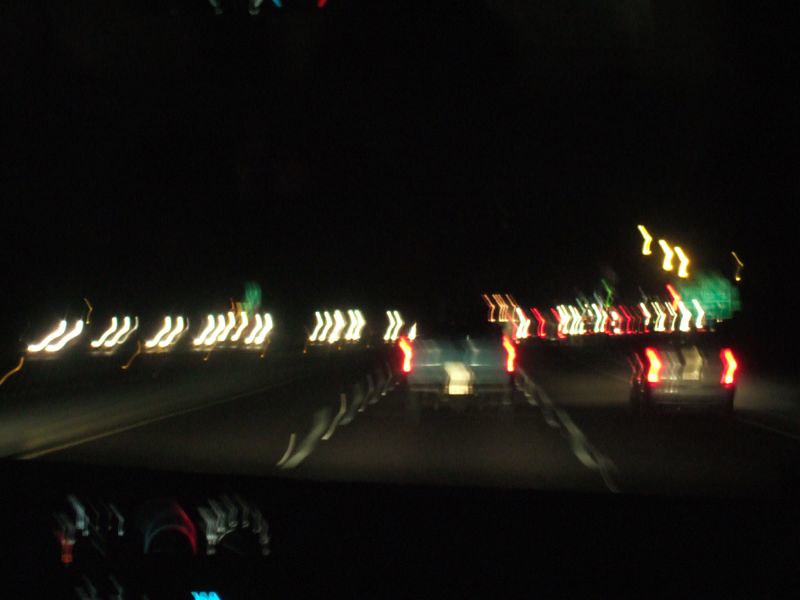This nighttime photograph, taken from inside a moving car on a highway, captures the blurred essence of motion. The dashboard is visible, with several illuminated gauges: one lit up in light blue, another in white, a third in blue and red, and a fourth displaying illuminated white numbers, though they are blurred. An LCD screen, glowing cyan, adds to the array of interior lights. Outside, the road is flanked by white lines and is dark gray to black in color. In the distance, a blue truck with a blurry license plate and red brake lights trails in front, while a sedan with rear lights illuminated travels to the right, possibly champagne-colored. Wispy streaks of white, red, pink, brown, and golden lights dance across both sides of the image, complemented by green splotches. The dark sky above adds to the atmospheric nighttime scene, accentuating the motion-blurred effect created, likely due to a bump on the road.